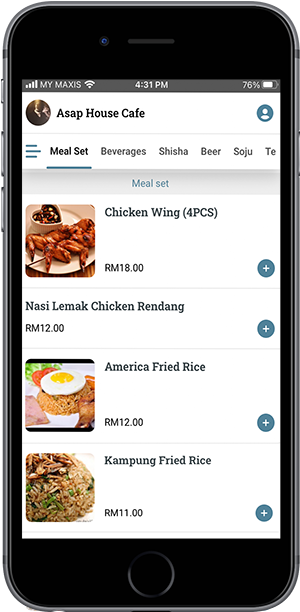This image captures a detailed screenshot of a smartphone displaying a webpage, outlined by the phone's frame, with distinct black borders at the top and bottom and visible gray buttons on the left side. 

At the very top of the screen, a thin gray status bar features several icons and indicators: on the left, the signal strength icon followed by the "My Maxis" network label; in the center, the current time displayed as 4:31 PM alongside the Wi-Fi signal icon; and on the right, a battery icon showing 76% charge.

Below the status bar, the webpage itself is set against a white background. Positioned to the left is a circular image of a man in a suit and white shirt, labeled "ASP House Cafe." To the right of this image is another circle with a generic person icon. Directly beneath this header is a white text box followed by a navigation bar featuring three horizontal bars labeled as the menu set, including sections for beverages, shisha, beer, soju, and tea.

Below the menu categories, the page lists several food items accompanied by images and pricing details:

1. A white plate of chicken wings with a brown dipping sauce in a heart-shaped container labeled "Chicken Wings (4 pcs), RM 18.00." To the right, a blue circle with a white plus sign invites the user to add the item.

2. The second item is "Nasi Lemak Chicken Rendang," priced at RM 12.00, also accompanied by a blue circle with a white plus sign for selection.

3. An image of a bowl of rice topped with a fried egg represents "American Fried Rice," priced at RM 12.00, with a blue circle and white plus sign to its right.

4. The final menu item depicted is "Kung Pong Fried Rice," featuring brown rice garnished with greens, priced at RM 11.00, also paired with a blue circle and white plus sign for adding the item to the order.

This succinct yet comprehensive snapshot captures both the functionality and visual details of the smartphone interface and the specific webpage content.